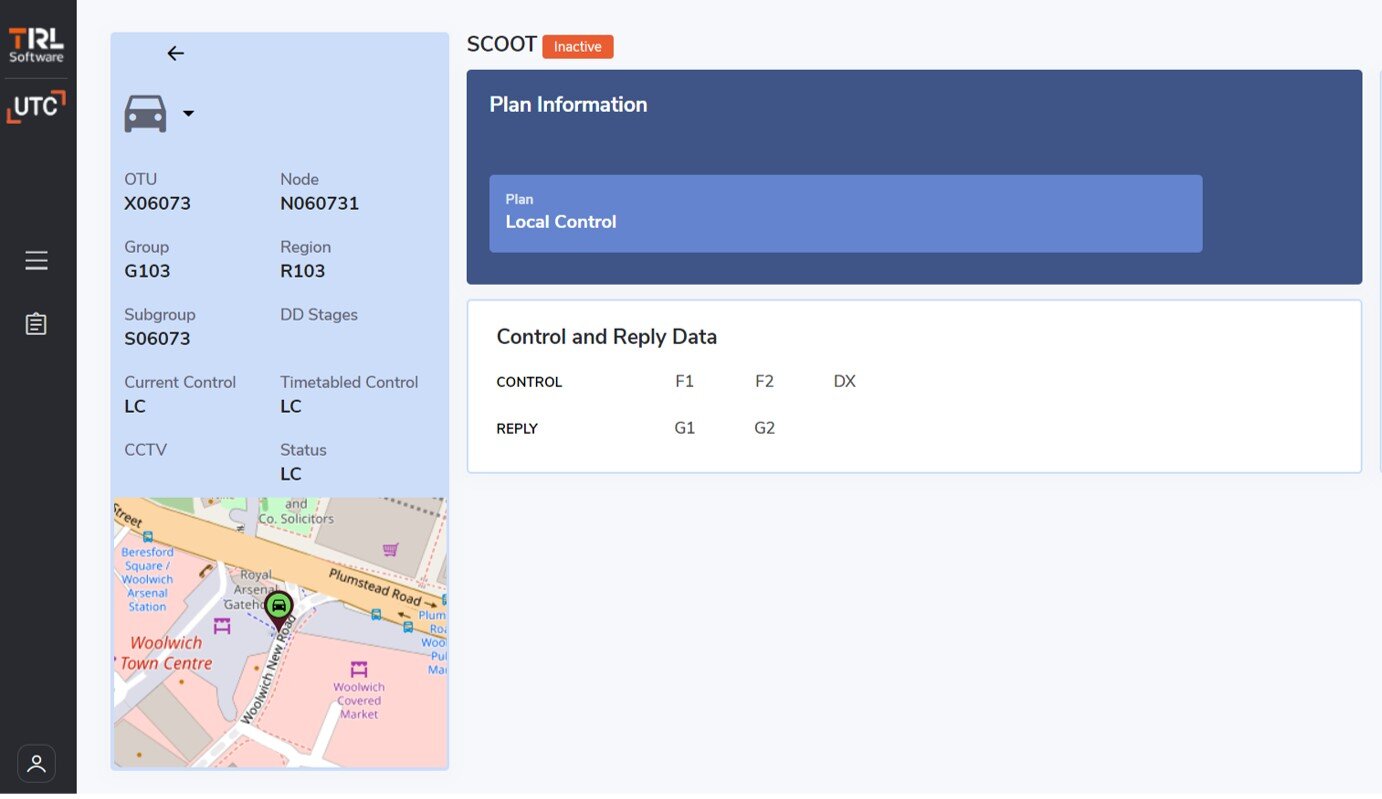This image depicts a detailed interface of an application, possibly related to traffic management or urban planning software. On the left-hand side, there is a vertical navigation bar with different icons and labels. At the top, the header displays the "TRL Software" logo, where the "T" is highlighted in orange, followed by a horizontal white line beneath it. Below this, another logo appears, featuring the letters "UTC" surrounded by orange L-shaped corners. Further down the vertical bar, a hamburger menu icon consisting of three stacked lines can be seen. Underneath the menu, there is an icon resembling a clipboard or a document. At the bottom of the vertical bar, a "My Profile" icon is present.

Adjacent to the vertical bar on the right side, there is a vertical rectangular information section displaying various data. This section includes labels such as "OTU," "XO6073," "node," "group," "region," "subgroup," "TD stages," "current control," and "timetable control," all within a light blue square.

Beneath this data section, a map is visible which specifically shows Plumstead Road. The streets are depicted in white, major streets in yellow, and the buildings or occupied areas in red.

To the right of the map, there is a darker blue box labeled "SCOOT inactive, plan information," with white text. Within this box, there is a thinner, lighter blue section for "plan local control," also with white text. Below this section, a white background area contains the text "control and reply data" in black, along with "control," "reply," "F1," "F2," "DX," "G1," and "G2."